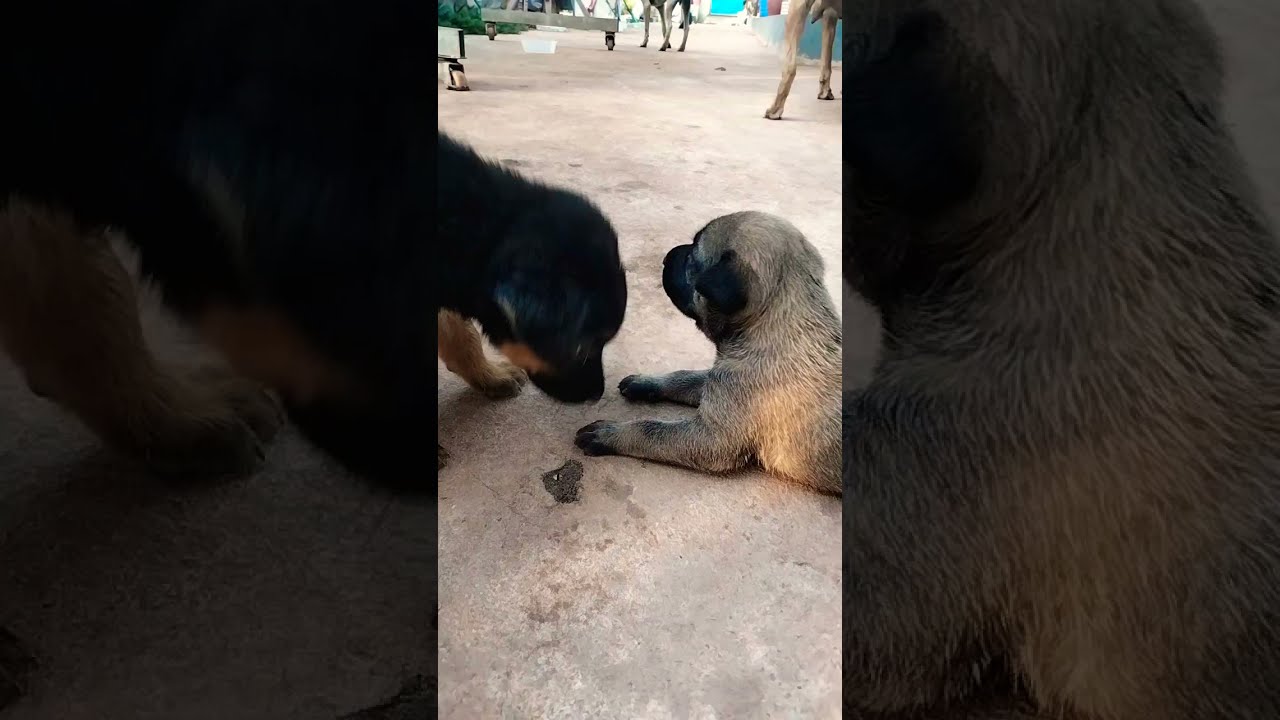The image captures a detailed scene featuring two dogs on a brown and gray concrete floor. On the left side of the image is a black and brown dog, standing partially inside a vertically-oriented rectangular frame. This dog has a black head and ears, with golden brown cheeks, and is looking down at the ground. On the right side, a beige dog with a black nose, ears, and paws is laying down, appearing wet and possibly dirty. This dog is positioned within a similarly oriented rectangular frame. Animal legs, thin and beige, are visible near the top of the image, indicating the possible presence of other dogs in the background, as if in a dog kennel or rescue setting. Additionally, a brown object is situated next to the reclining dog on the right. The overall lighting differentiates the center image, which is bright and clear, from the darker, shadowy side images.